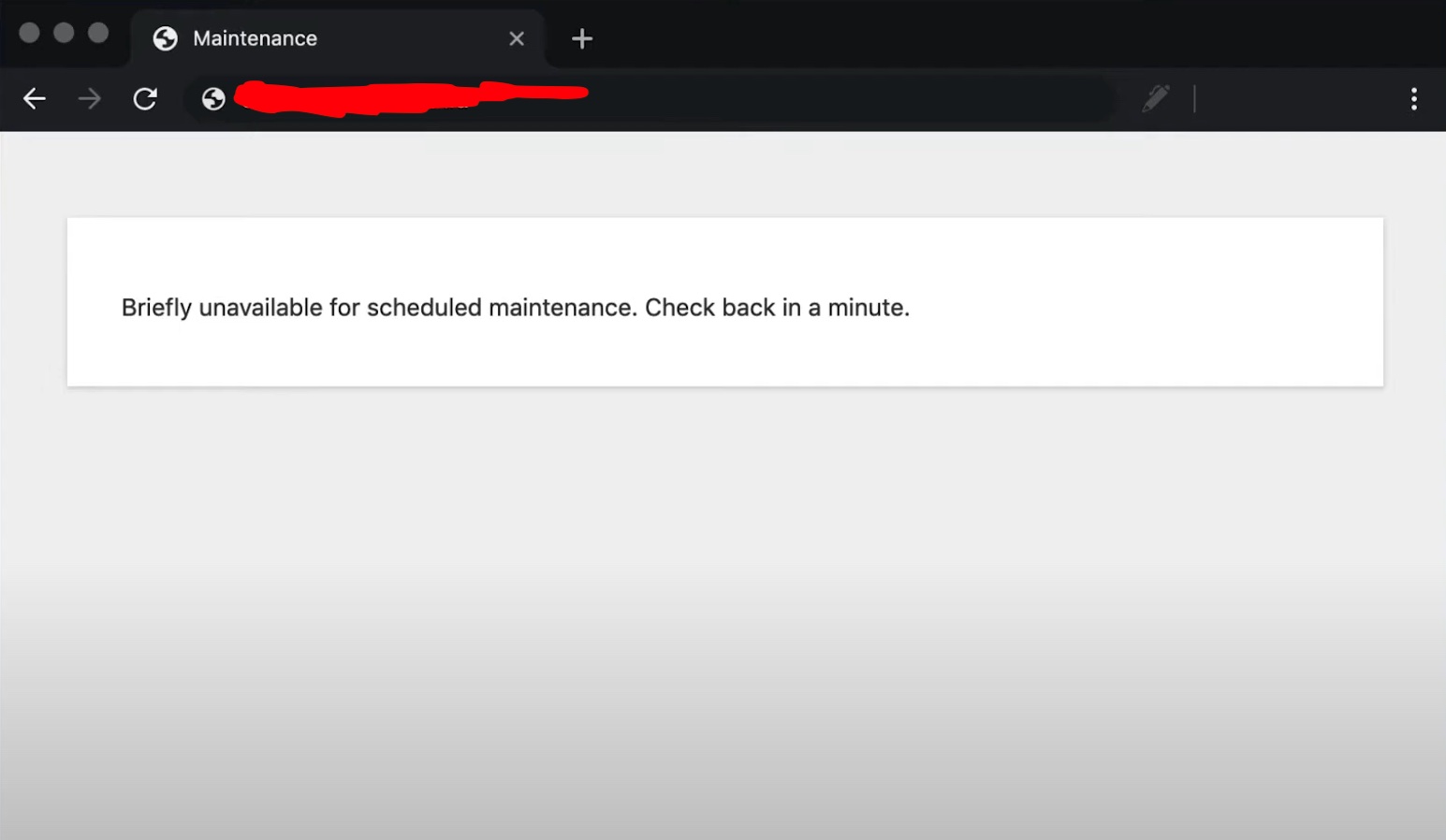The image showcases a web browser displaying a webpage that is under scheduled maintenance. The website's URL is obscured with red scribbles, effectively hiding any identifiable information. At the top of the page, the word "Maintenance" is prominently displayed alongside an icon resembling a welding torch, symbolizing repair work.

In the browser tab itself, there is an 'X' button in the top right corner to close the current tab, and a '+' sign to open a new one. The browser's interface features a dark theme. The URL address bar includes several icons: a back arrow for navigating to the previous page, a refresh button for reloading the page, an icon indicating the website's security status, and a three-dot menu icon on the far right representing additional browser options.

The main content area of the webpage has a white background with black text that reads: "Briefly unavailable for scheduled maintenance. Check back in a minute." This message indicates that the website is temporarily down for routine upkeep and should be accessible shortly.